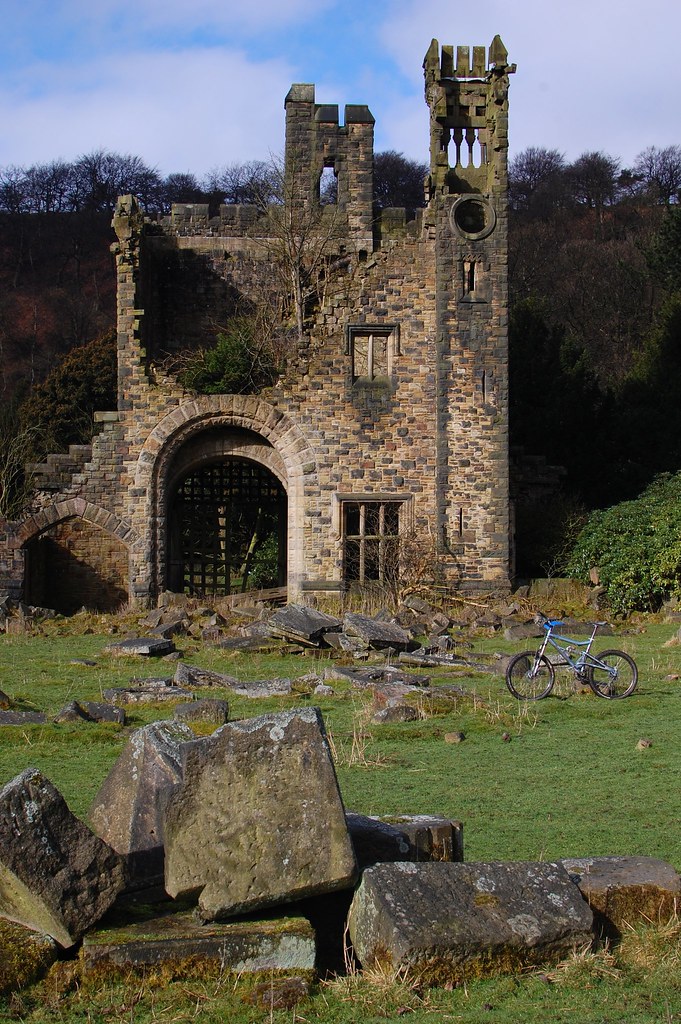The photograph captures a dilapidated, medieval stone castle set against a cloudy sky with light blue and gray hues. The castle appears crumbling and weathered, with a variety of stone colors including light brown, dark brown, red, and charcoal black. In the center-left of the image, significant structural damage reveals the castle's interior, through which a tree has started to grow. The foreground is littered with rubble—ranging from light brown to gray stones—intermingled with patches of green grass and moss.

A prominent feature of the left side is an archway with a dark steel gate below, and two windows, one on each of the bottom and second floors, are visible to the right side of this archway. To the right of the photograph, a structurally sound tower stands, characterized by its aged, multi-colored brickwork. 

In front of the castle, near the center-right of the image, sits a modern, light blue bicycle surrounded by scattered stones and more greenery. Distant trees with dark red and black tints shadow the background, adding to the eerie, abandoned atmosphere. The entire setting appears to be within a small valley, with the green leaf trees and a hill subtly visible behind the castle.